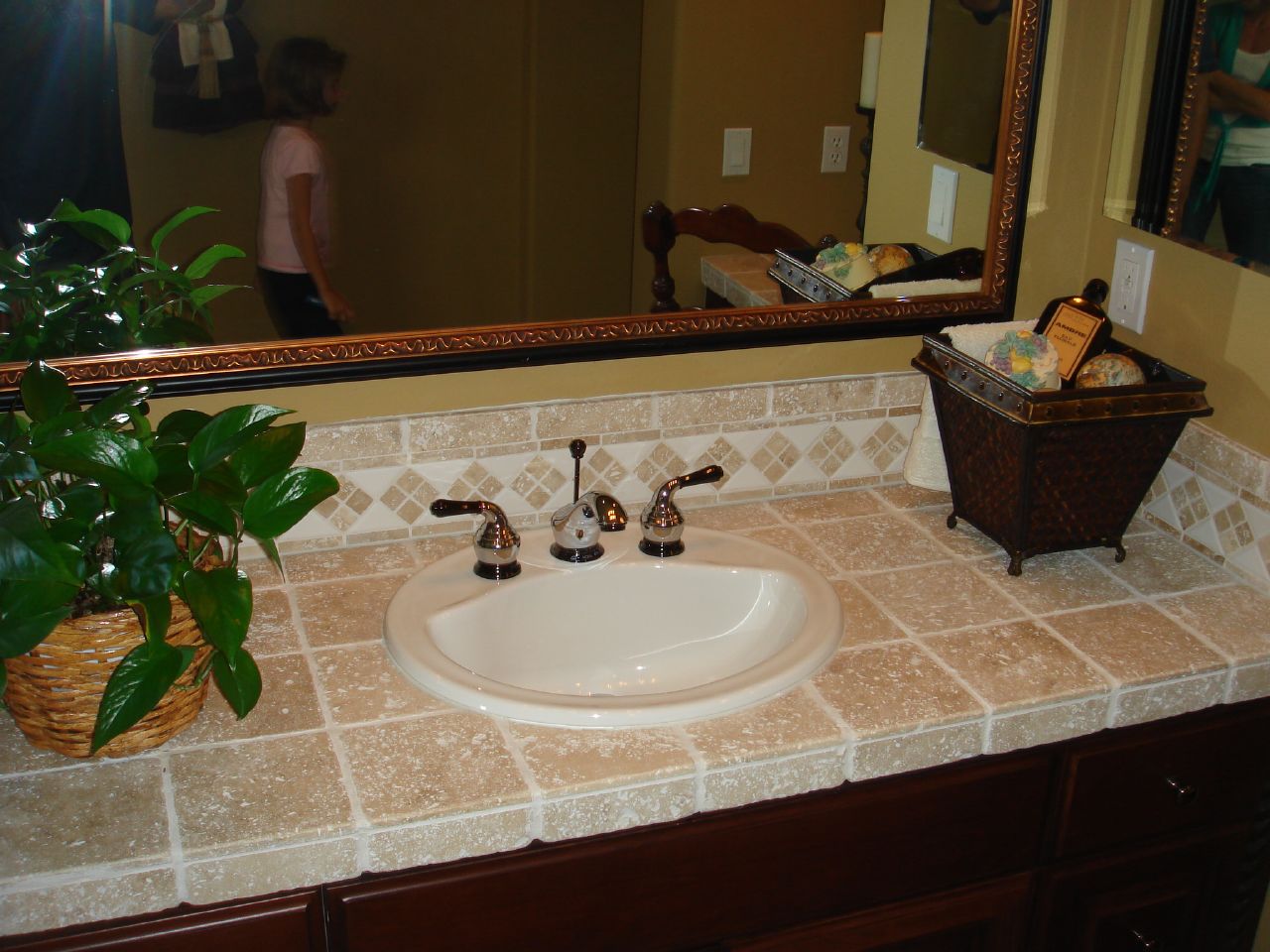The image depicts a kitchen sink positioned prominently in the center. The photograph has a slightly wider-than-tall aspect ratio, around 20-30% wider. The countertop, visible from the lower left corner to approximately a quarter of the width from the right edge, is tiled with medium brown squares speckled with white, complemented by off-white grout lines. 

The sink, centrally located, appears impeccably clean and off-white, practically glowing under the light. It features a pair of gold faucet handles oriented to the left and right, with a matching gold faucet spout. 

To the right of the sink, there is a square-shaped brown basket, which widens towards the top and stands on four small peg legs. On the left side of the sink, a plant in a light brown wicker basket adds a touch of greenery. The plant's leaves are narrow, shiny, and distinctly green, suggesting it might be an artificial decoration.